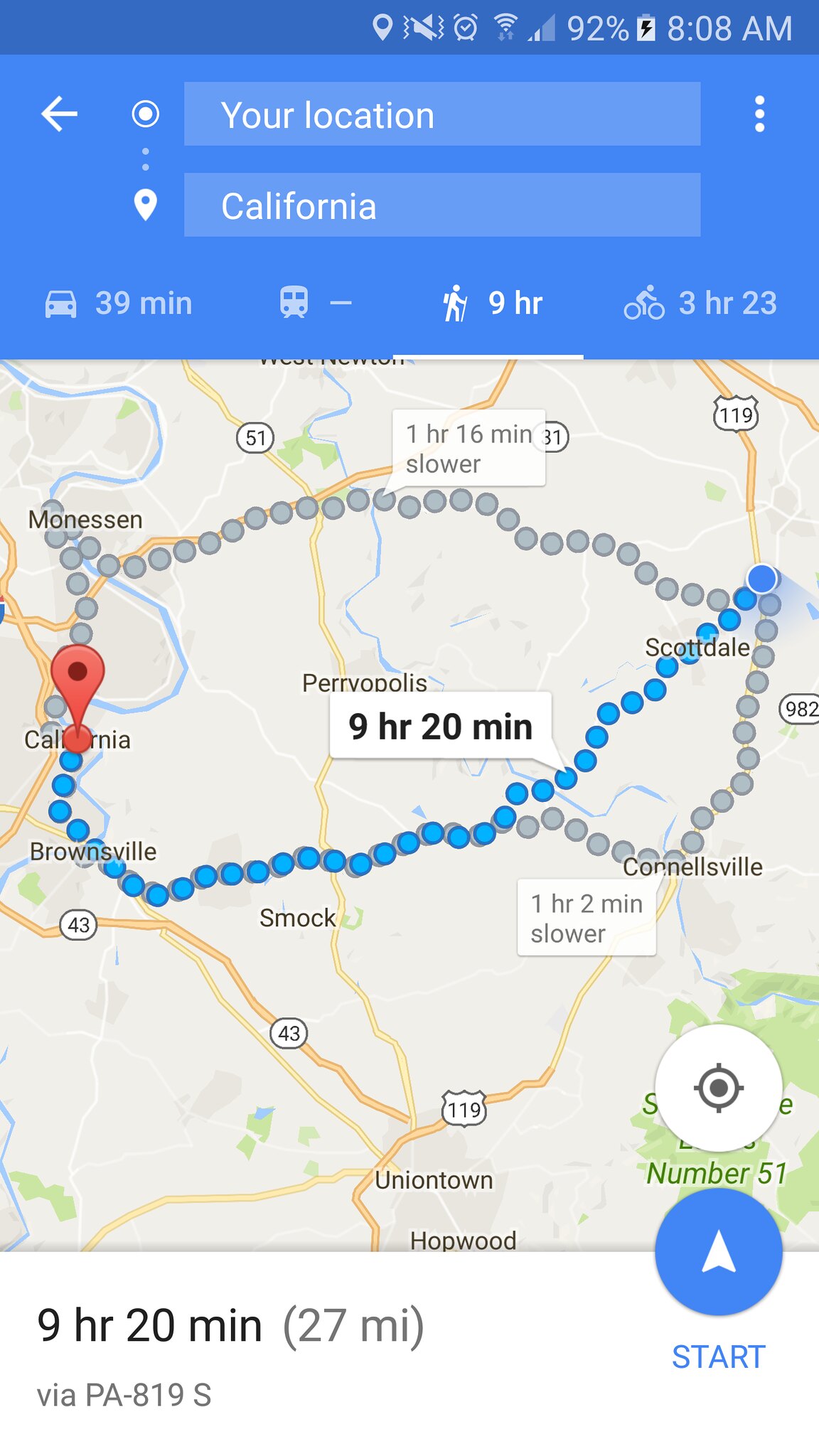This is a detailed screenshot from a map application on a cellphone, displaying various features and navigation options. At the top of the image, there is a dark blue status bar showcasing essential icons such as the current time, battery percentage, Wi-Fi signal strength, and other symbols. Just beneath this, a light blue field houses the search bar. Within this field, on the left side, is a left-pointing arrow symbolizing the return function, while on the right side, three vertical white dots represent the options menu. The search bar indicates a search for locations in California.

Directly below the search bar, there is a row of transportation mode icons: a car, a train, a hiker, and a bicycle, with the hiking symbol being currently selected. The main map area depicts a non-satellite, standard layout with visible roads and route options. Two primary routes are illustrated: the fastest route is marked with blue dots, while alternative, slower routes are shown in gray. One of the gray routes deviates slightly from the main blue-dotted path.

At the bottom of the map, a white information panel displays the estimated travel time and distance for the selected hiking route. It indicates "9 hours 20 minutes" and "27 miles," with an option to start the navigation prominently shown.